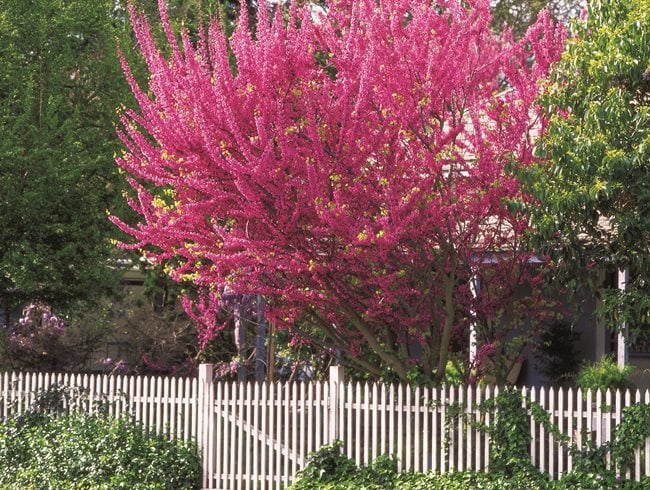The photograph captures the front view of a house, partially obscured by a vibrant floral display. Dominating the scene is a tree with abundant pink blossoms, which cover much of the branching structure. This main tree stands prominently in front of a white picket fence, which features a gate section and is complemented by green shrubs along its length, except at the gate opening. Vines trail along the right side of the fence, adding to the lush greenery. To the right and left of the blossoming tree are other trees with green leaves, forming a verdant canopy that surrounds the area. Although the house is largely hidden by the trees, parts of it are visible, revealing a light-colored roof and a porch with white pillars. The sunny daytime scene is suggested by light reflecting off the roof, casting a serene glow over the entire setting.